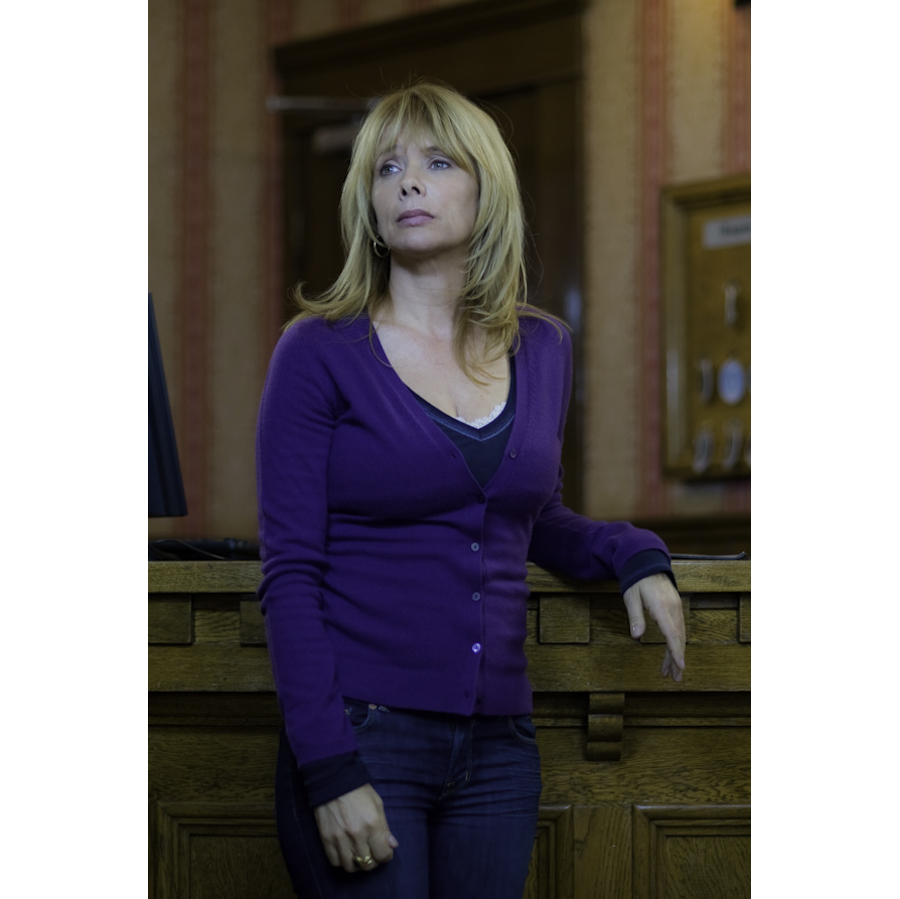In this color photograph, we see a woman with long blonde hair, falling just past her shoulders, who appears to be in her mid-50s or slightly older. This actress, recognizable from her work in the 1980s and known to have a sister currently active in acting, is leaning against a wooden bar or high table made of honey-colored wood. She has striking blue eyes and wears a coordinated outfit comprising a blue v-neck t-shirt and a blue buttoned-up cardigan, along with jeans. A hoop earring adorns her right ear, while the left is obscured by her hair. A white lace undergarment subtly peeks from beneath her top. The actress's right arm rests at her side, displaying a ring on the middle finger, while her left arm is draped over the table, her hand hanging slightly below. Her gaze is directed off to the left (our right), evoking a contemplative expression. The background features red and white striped wallpaper and a wooden door frame visible to the right, along with a wall-mounted display, possibly featuring cell phones.